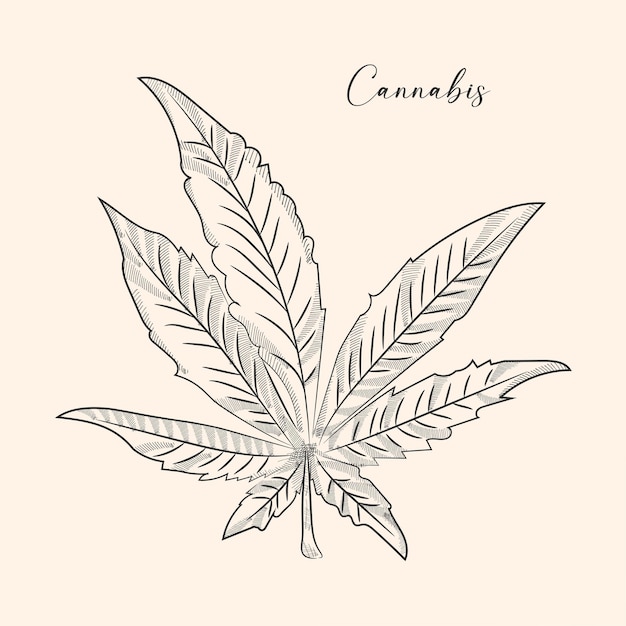The image showcases a meticulously detailed drawing of a cannabis leaf on creamy, off-white paper. At the top right corner, the word "cannabis" is elegantly inscribed in cursive with fine black or gray ink. The focal point of the piece is the large cannabis leaf itself, drawn with remarkable precision, possibly using pen or pencil. The leaf features seven distinct points and a small stem, each element intricately shaded to highlight the veins and texture. The overall style is simple yet sophisticated, with well-defined shadows and a feminine touch in the lettering. The absence of color and additional text emphasizes the clarity and craftsmanship of the black-and-white illustration.